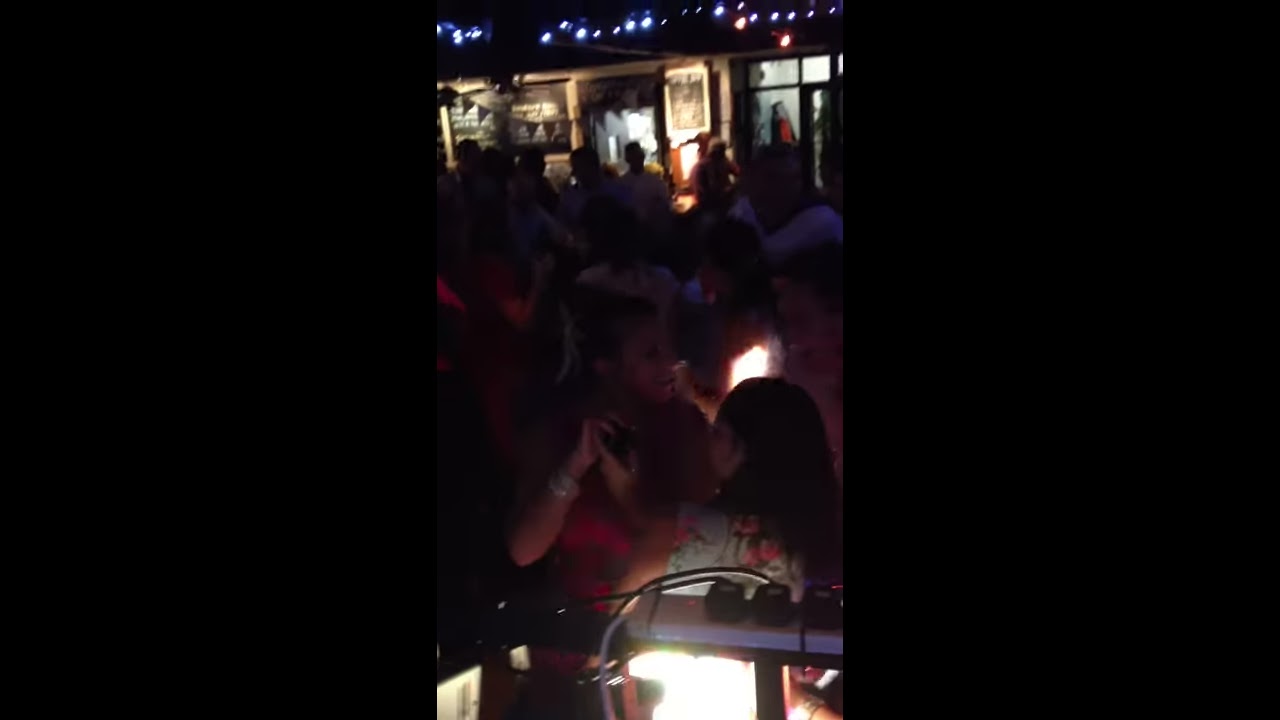The vertical cell phone image captures a dimly lit nighttime party scene, bordered by black spaces on the left and right. The camera is positioned slightly above the revelers, providing an elevated view of a crowd engaged in dancing and merrymaking. In the foreground, there is a light source that highlights a small area near the camera. Approximately 50 feet in the distance stands a possibly residential building adorned with decorative lights along the roofline and small triangular flags hanging from a cord beneath the roof. Despite the darkness making it difficult to discern individual features, the joyful atmosphere is palpable, with people enjoying what seems like an outdoor celebration under the minimal but festive illumination.